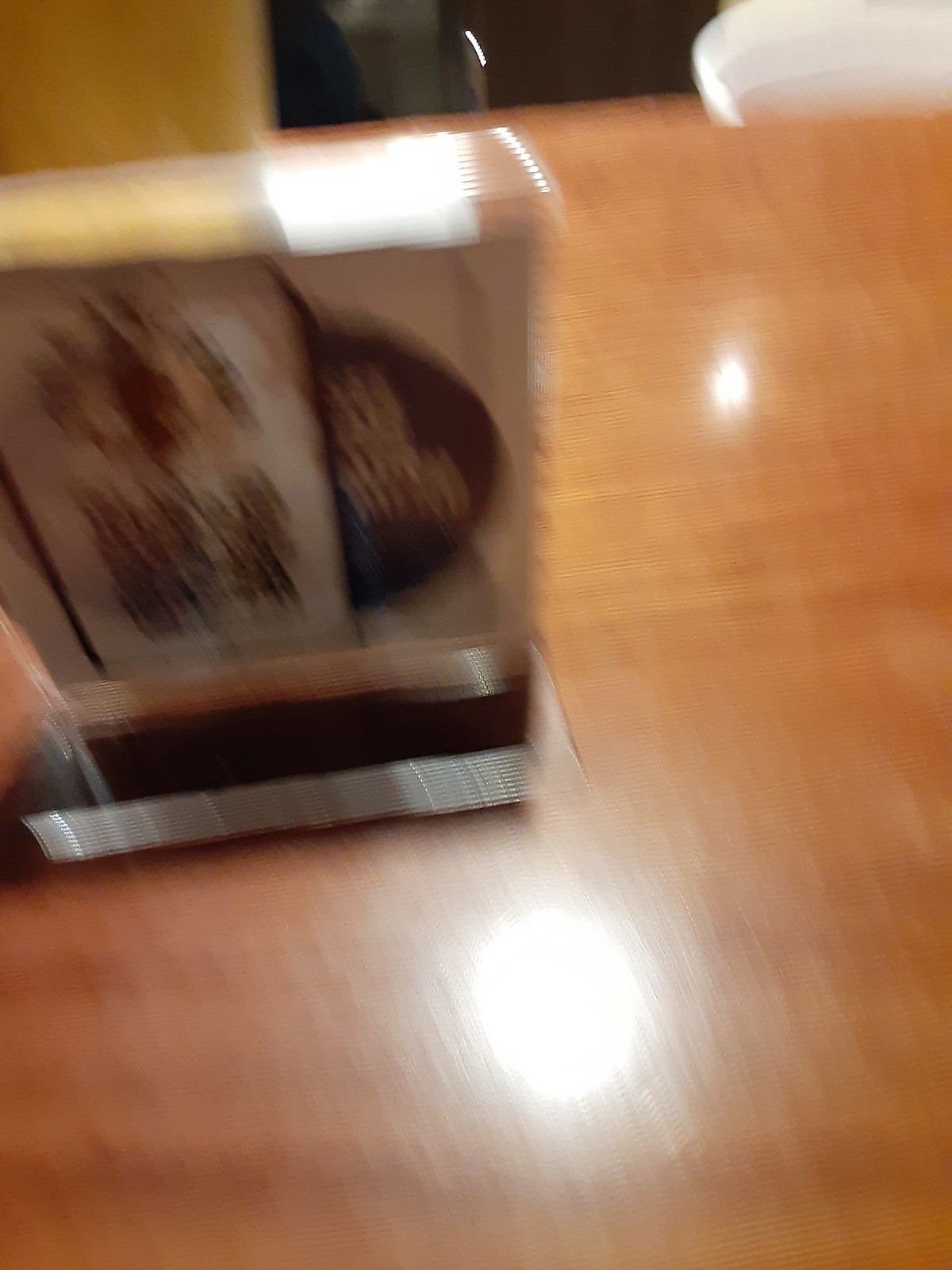This extremely blurry photograph primarily captures a medium to light brown wooden table, or possibly a wooden countertop, characterized by horizontal grain marks. The image is heavily out-of-focus, making it difficult to identify specific items. However, there's a rectangular object situated on the table, featuring a clear or silver rectangular base which is possibly transparent plastic. The object itself seems to be covered in plastic and has a combination of dark, silver, brown, and white within, with oblique streaks that suggest some form of text or design, possibly a menu, paperweight, or even a trophy. Reflections from lights above are seen as large and smaller light-colored circles at the bottom and upper right-hand quadrant. Additionally, there is a hint of a yellow item on the left and what might be the curved back of a white chair in the background.